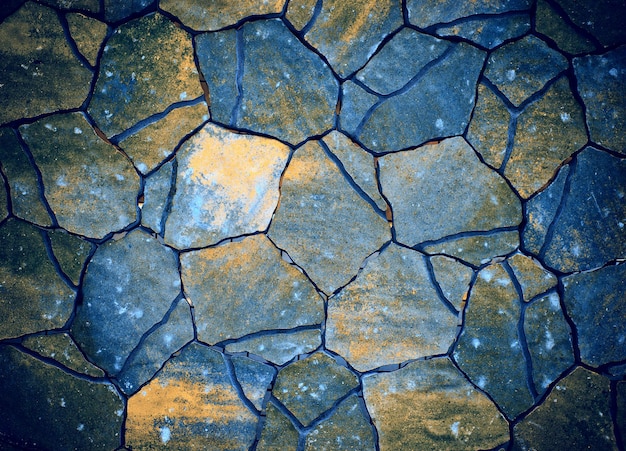The image depicts a rectangular stone pathway, approximately four to five inches wide and three to four inches high, composed of cracked stone tiles intricately pieced together. The tiles exhibit a rich palette of blues, grays, and hints of yellowish-brown, with at least three distinct shades of blue. The bottom pieces feature bright blue highlights, particularly noticeable just left of the center, while the center of the image displays a mildly dark blue tile. Yellow crystal-like specks are scattered across many of the top tiles, giving them a sparkling, almost golden appearance. A notable feature is a single blue scraped line that runs through most of the stones, adding dimension and texture to the surface. These lines vary in shape, some forming Y shapes, others curving at the corners, creating a dynamic pattern. The corners of the stonework appear darker and more defined, whereas the center lightens up. The tiles are laid flat and pressed against each other, some tightly fitted with bluish-gray mortar, while others are yet to be filled in, contributing to the pathway's intricate and textured aesthetic.